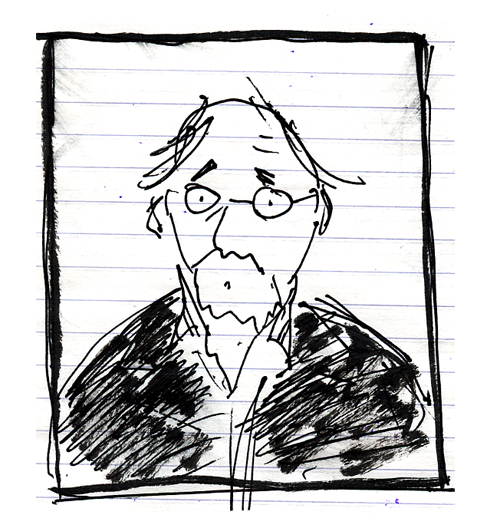The image is a digital drawing set against a white background with light blue lines imitating a lined drawing pad. Central to the image is a rectangular frame, outlined in black, creating a border that has been drawn repeatedly, giving it a duplicated, sketchy appearance. Within this frame is a crude and impressionistic drawing of an elderly, balding man with hair on the sides of his head. He sports round glasses and has dark, slanting eyebrows set in a worried expression. The man's face features a nose but lacks a defined mouth, while a mustache and beard are faintly visible. His clothing resembles a shirt with a V-neck and a collar, and there are scribbled black areas on the left and right sides of the shirt. The background also features smudges in the upper left and right corners.